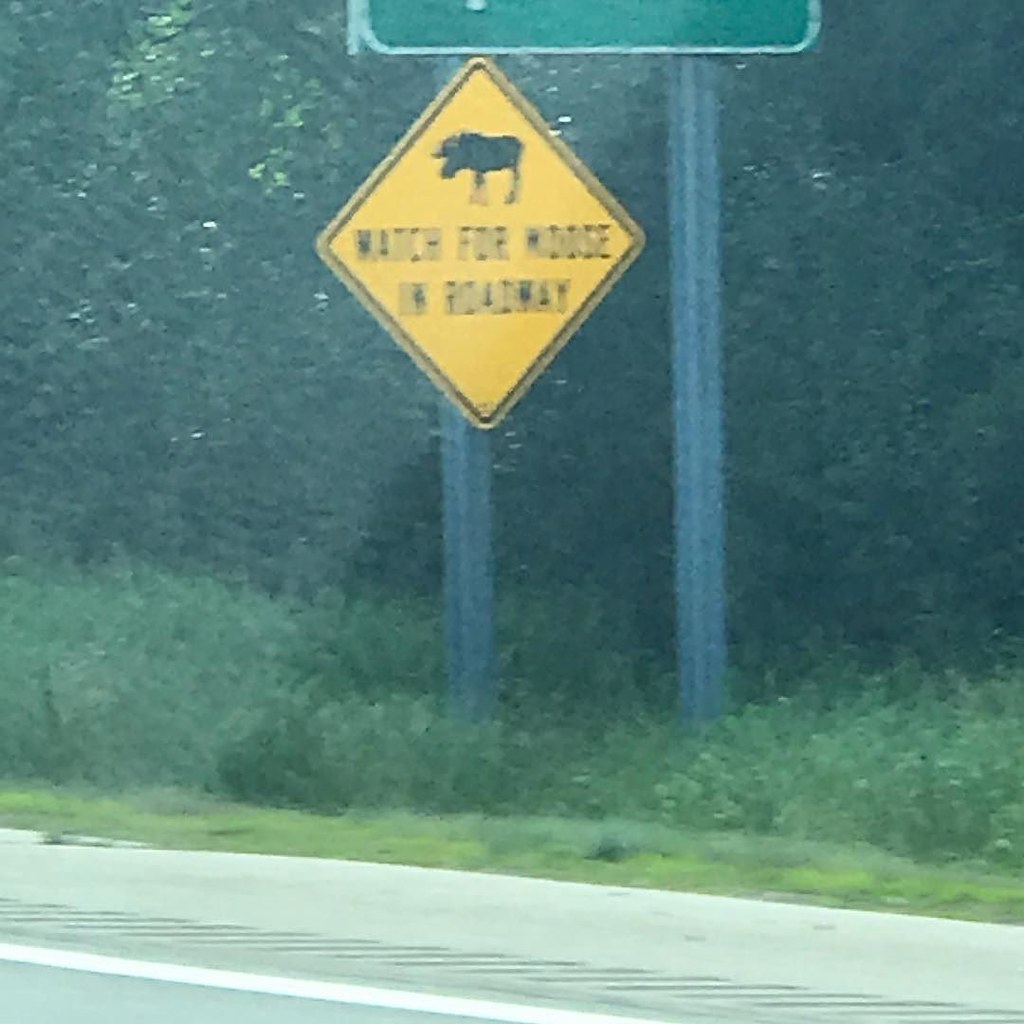A low-quality image captures a small yellow road sign on the side of a road, with a pictogram and text cautioning drivers to "Watch for Moose in Roadway." An image of a moose is prominently displayed above the warning. The sign is mounted on a slender pole, and to the left of the foreground, the road itself is partially visible, running diagonally from the lower right to the lower left corner. Dense woods can be seen lining the roadside, adding to the cautionary nature of the signage. Additionally, the bottom portion of a green exit sign protrudes from the top edge of the frame.